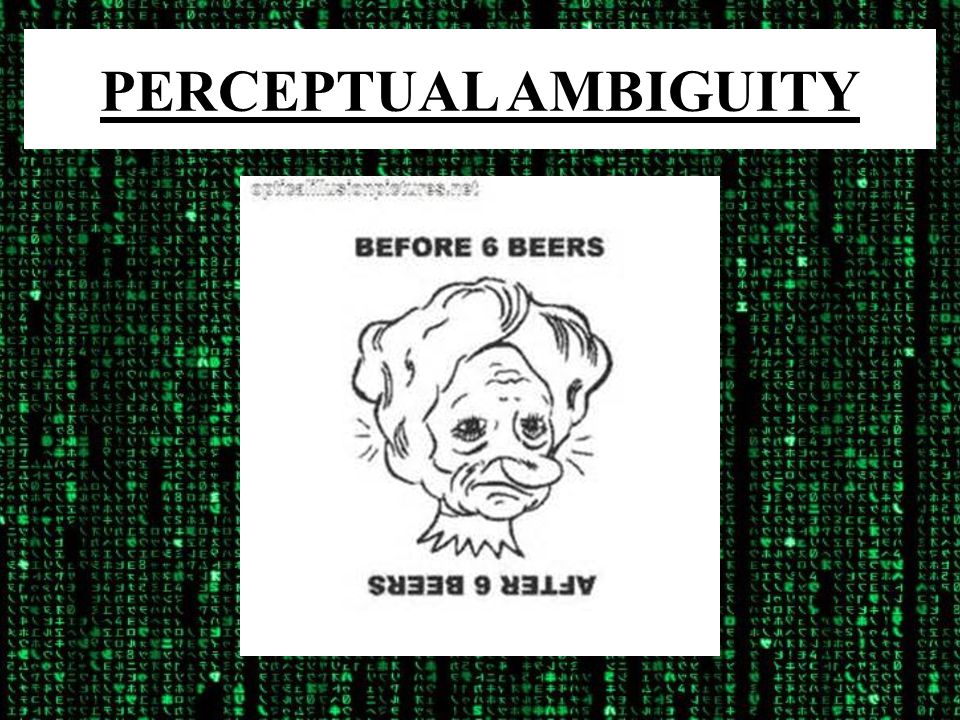This image, entitled "Perceptual Ambiguity," prominently features a white band at the top with the title in black underlined text. The background is reminiscent of The Matrix, with green cascading letters, including Japanese characters, forming a digital curtain effect. Below the title, there is a white square containing a dual-image. Initially, the image depicts an older, unattractive woman with the caption "Before Six Beers" above. However, "After Six Beers" is written upside down below, prompting viewers to flip the image. When inverted, the old woman transforms into a beautiful princess, illustrating a perceptual shift influenced by context. The entire composition plays on visual ambiguity, engaging viewers to explore different perspectives.